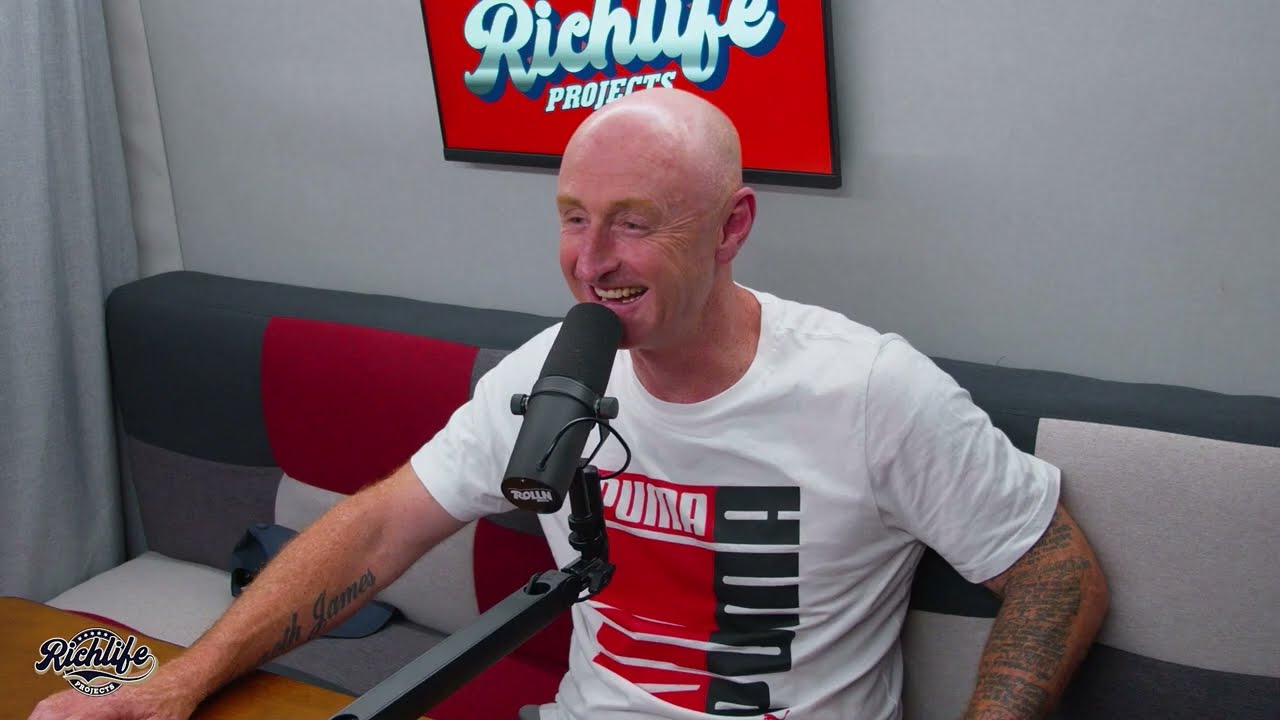The image depicts an older Caucasian man, likely a guest on a talk show or podcast. He is seated on a gray, patterned sofa adorned with blocks of red, white, and various shades of gray. Dressed in a white short-sleeve Puma t-shirt featuring the brand's name in red and black text, he sits in a room with gray walls. Above him is a red sign displaying "Rich Life Projects" in white and gray letters, trimmed in black. He is bald with faint eyebrows and has tattoos on both arms; a small one that appears to say "James" on his right arm and an intricate paragraph on his left arm. The man is smiling, revealing his teeth, and is speaking into a black microphone positioned on a brown desk in front of him. His right arm rests on the desk while his left arm is bent out of view. In the bottom left of the image, the "Rich Life Projects" logo can also be seen on a wood structure, and to his side on the sofa sits a hat.